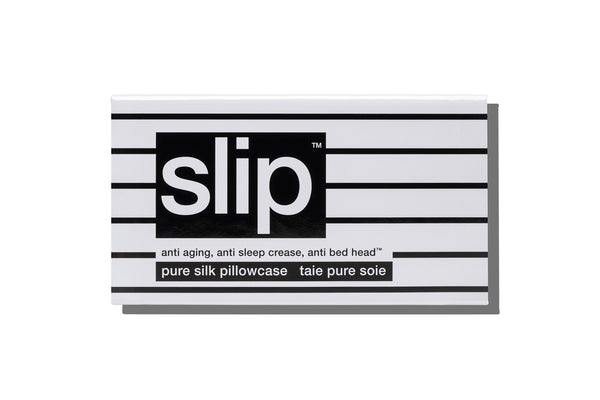The image is of a product tag or business card shaped in a small, elongated rectangle with a 3D appearance due to a subtle drop shadow against a light gray background. The card itself is light gray with six bold, horizontal black stripes creating an alternating pattern with the background. On the left side of the card, slightly above the center, there is a prominent black rectangle featuring the word "SLIP" in thick white letters with a trademark symbol (TM) at the top right. Below this, a longer, skinnier white rectangle contains the phrases "anti-aging," "anti-sleep crease," and "anti-bed head," all in black text with a trademark symbol next to them. Further below, another black rectangular box holds the words "pure silk pillowcase" and "Tai Pure Soe" in thin white text. The card's border features a slightly darker gray shading along the bottom and bottom right edges, accentuating the design.